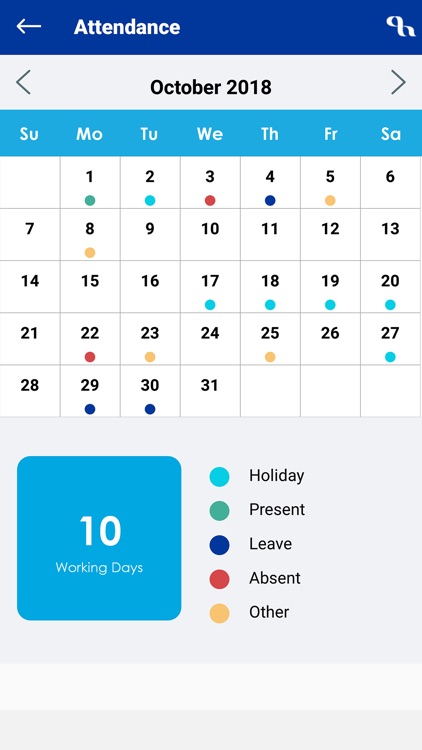The image is a detailed calendar layout for October 2018. In the top right-hand corner, there is a diagonal infinity symbol in white, accompanied by arrows pointing left and right. Below it, the text "October 2018" is displayed.

Across the top of the calendar, there is a horizontal blue bar listing the days of the week: Sunday, Monday, Tuesday, Wednesday, Thursday, Friday, and Saturday. The calendar follows a standard format, with each day of the month laid out in a grid.

Several days within the month have colored dots, each indicating a specific status:
- Light blue circle for holidays
- Green circle for present days
- Dark blue circle for leave
- Red circle for absences
- Yellow circle for other reasons

The marked days are as follows:
- Green on the 1st
- Light blue on the 2nd
- Red on the 3rd
- Dark blue on the 4th
- Yellow on the 5th and the 8th
- Light blue on the 17th, 18th, 19th, and 20th
- Red on the 22nd
- Yellow on the 23rd and 25th
- Light blue on the 27th
- Dark blue on the 29th and 30th

At the bottom of the calendar, a blue square indicates "10 working days" in white text. The background is predominantly white, providing a clean and clear presentation of the calendar details.